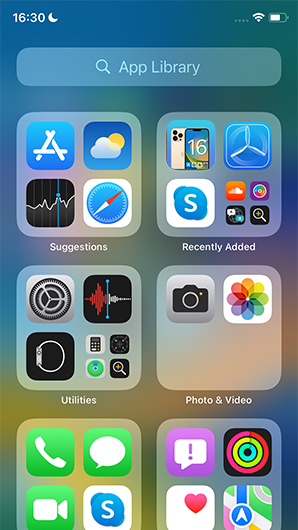This is a detailed screenshot from a smartphone. In the top left corner, the time is displayed as 16:30 along with a moon icon indicating night mode or nighttime settings. On the top right, there are four horizontal dots, a signal icon, and a battery icon that appears to be around two-thirds full. Below this, there's a search bar with a magnifying glass icon and the text "App Library." Underneath the search bar, there are six light gray-colored squares, each containing a maximum of four icons.

In the top left square, labeled "Suggestions," there's an icon of the Sun with clouds against a blue sky, an icon of a compass below it, another icon with a graph to the left of the compass. The square in the top right corner contains a smartphone picture with the Skype logo, and the label underneath reads "Recently Added."